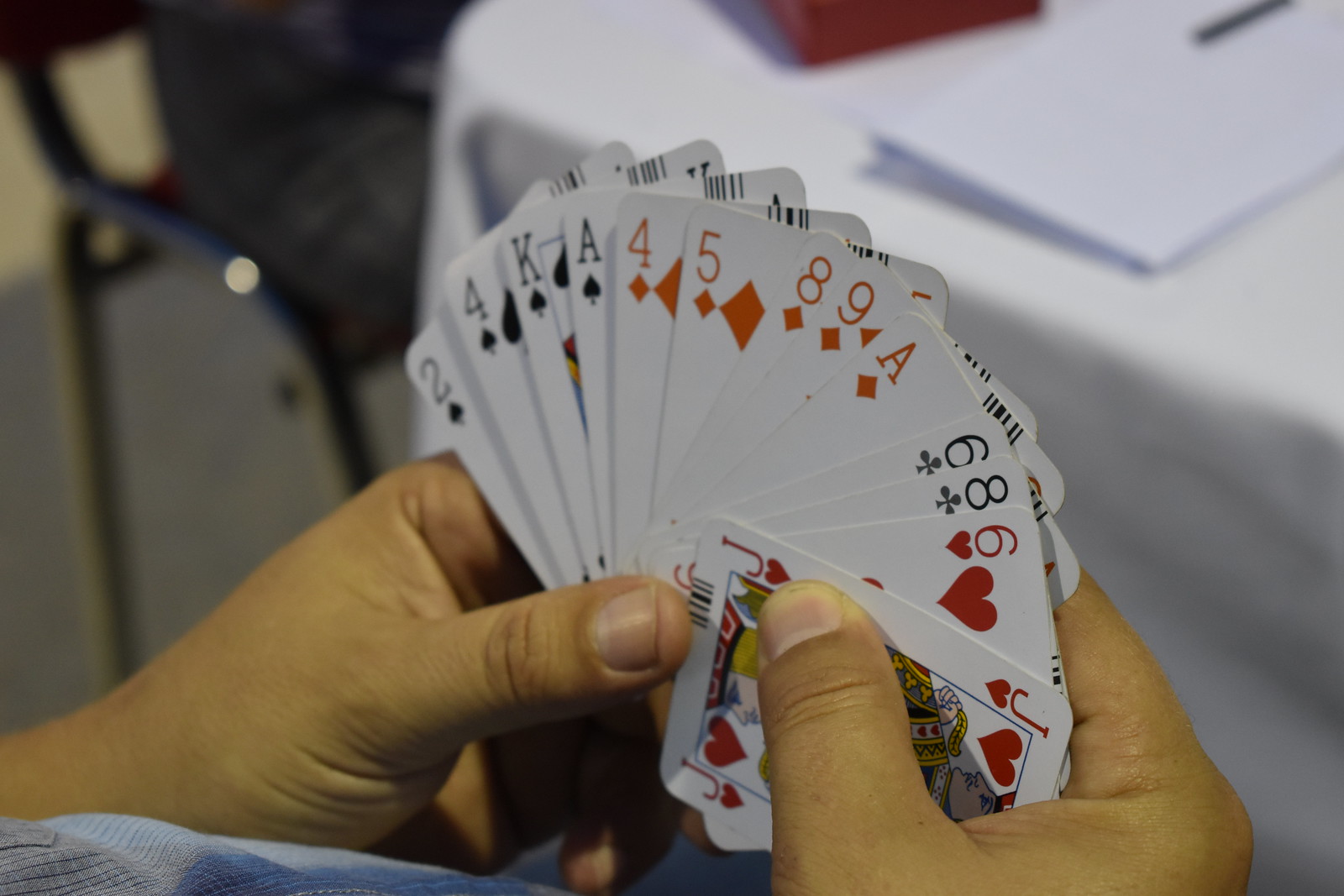A detailed and focused photograph depicts a person's hand holding a fan of thirteen playing cards. The hand shows a diverse collection of cards, including two aces—one black and one red—as well as various other cards such as sixes, eights, a two, jack, king, and four. These colorful cards stand out sharply against the blurred background. The setting appears to be a card game at a table covered by a white tablecloth. Adjacent to the hand holding the cards, a chair is partially visible on the left side of the frame. On the table, there's a piece of paper and a small glimpse of a red box. The person's hand and the playing cards are the main subjects and are in perfect focus, creating an appealing contrast with the softly blurred background that includes the table and its accessories. This simple yet engaging digital image captures the essence of a quiet moment in a card game.